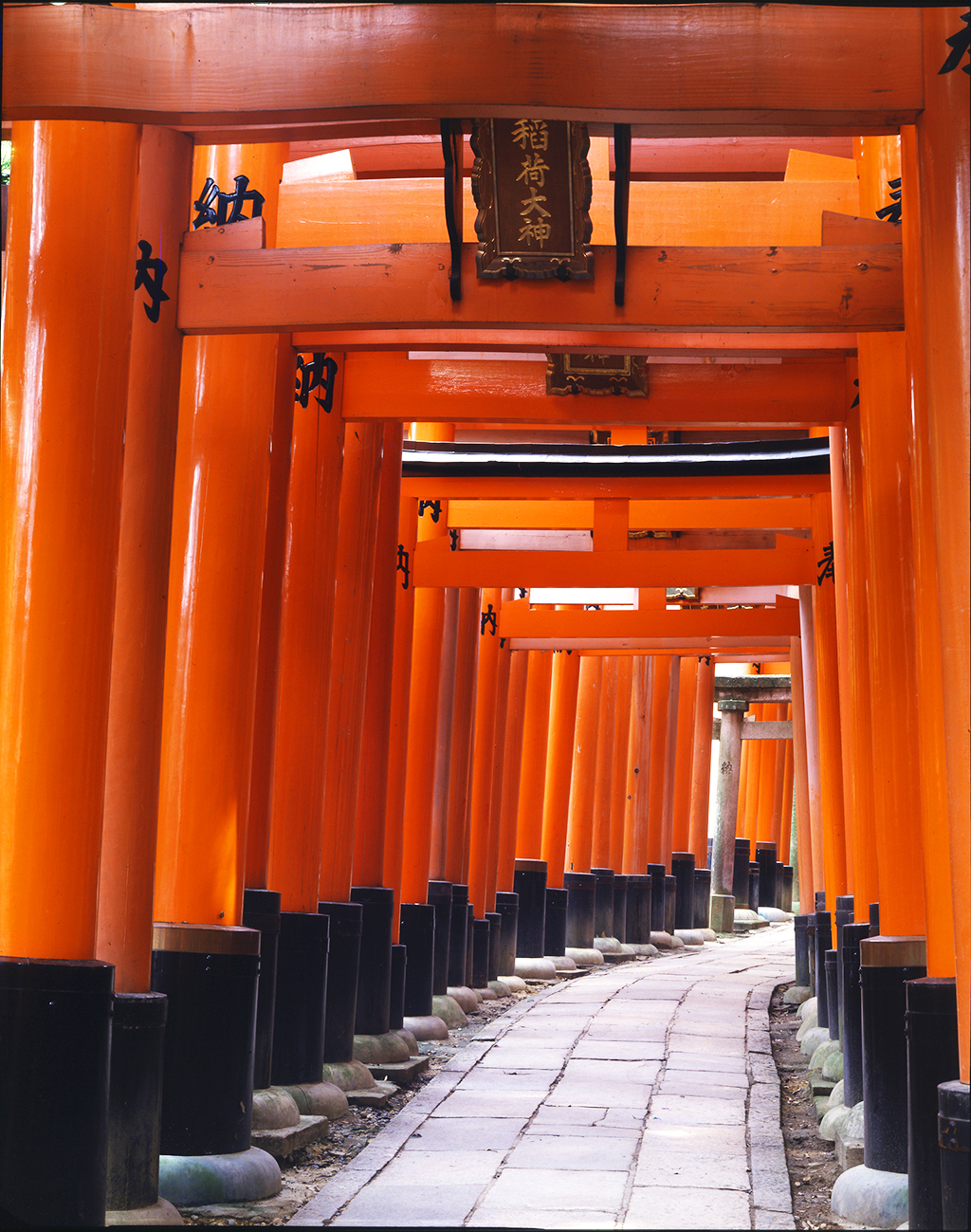This image captures the perspective of walking through a famed Japanese shrine entrance, marked by an impressive series of tall, reddish-orange torii gates. Each gate features black supports at the base, transitioning into the vivid orange hue. Adorning the gates are plaques with Japanese symbols, traditionally believed to bring prosperity or good fortune. The pathway beneath the arches is composed of weathered, gray, and white stone, adding to the aged charm of the shrine. As the path extends into the distance, the torii gates gradually recede in size, ultimately leading to a distinctive white gate at the far end, which notably lacks the symbolic signage seen on the others. This serene and visually striking corridor exemplifies the spiritual and architectural beauty of Japanese temple entrances.